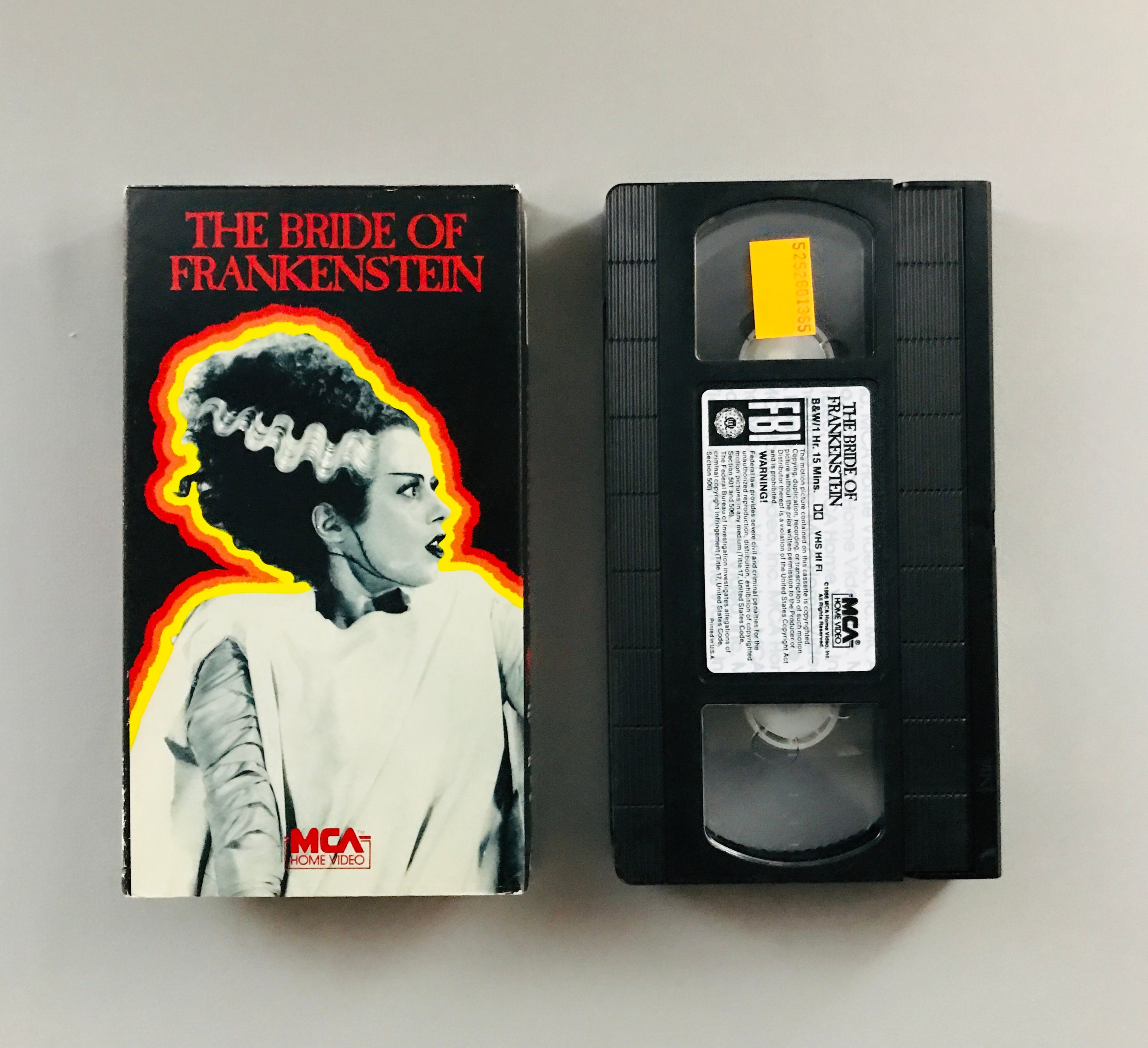This photo showcases a vintage VHS tape and its case, both lying flat on a white table. The black VHS case, positioned on the left, features a striking black-and-white image of a woman with tall, curly hair and a distinctive white streak, characterized as the Bride of Frankenstein. This image is encircled by a vibrant border of yellow, orange, and red. At the top of the case, "The Bride of Frankenstein" is printed prominently in red text, and the bottom bears the MCA Home Video logo. Adjacent to the case, on the right, resides the black VHS tape. The tape features clear windows that reveal the film inside, and it carries a centrally-placed white and black sticker label that again reads "The Bride of Frankenstein" along with another MCA logo and smaller text, including an FBI warning. Additionally, a yellow rectangular price tag with black lettering adheres to the upper clear window of the tape.